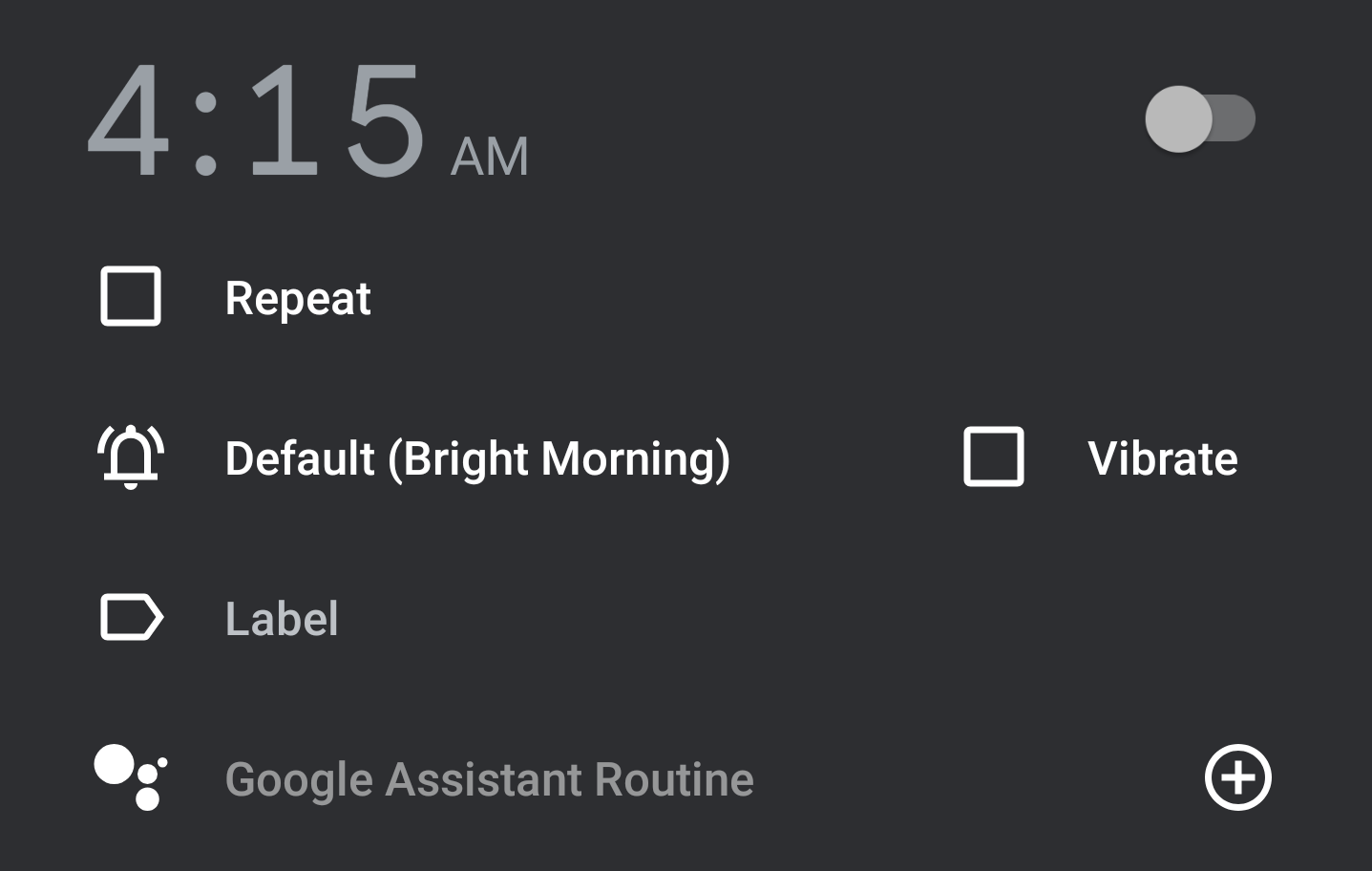This image captures a settings panel on a smartphone screen, featuring options related to Google Assistant. The background has a subtle color, though the specific hue isn't clearly described. 

In the upper left-hand corner, "4:15 AM" is displayed in a gray font, indicating the current or set time. To the upper right, there is a toggle switch, which is currently set to the left position, signaling that it is off.

Beneath the time, there are four configurable options:
1. A square icon labeled "Repeat" in white font, accompanied by a bell icon. This option is marked as "Default" with the specification "Bright Morning".
2. A box with a triangle on the right side, labeled "Label".
3. A series of circles denoting a "Google Assistant routine".
4. To the right of the "Default" label, there is another white box followed by the word "Vibrate".

In the lower right-hand corner, a circle with a plus sign at its center is visible, likely for adding new settings or alarms.

This screen is indicative of a settings interface within a smartphone, where the user is customizing their Google Assistant configurations. Although the alarm feature is currently off, the user appears to be in the process of setting it up to their preferences.